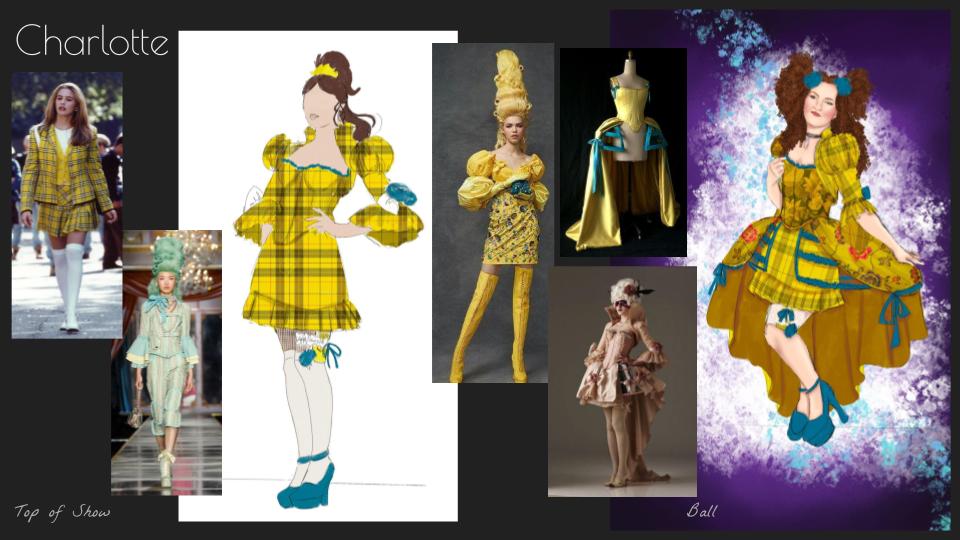The image displays a collage themed around a show titled "Charlotte Top of Show," prominently featuring a girl on the far left dressed in a vintage-style outfit. She dons a yellow plaid skirt and jacket with black stripes, a yellow vest, a white shirt, and long white stockings paired with white shoes. Her long brown hair frames her face, enhancing her classic look. Adjacent to her, several renditions of similar outfits are showcased, including a paper doll version of her attire. One version features a girl mimicking the outfit with long yellow boots and her hair styled in a tall bun. Another rendition displays a girl in a pink dress with a similar vintage essence, while a cartoon variant illustrates a girl with very curly hair, maintaining the overall style. The composition blends real-life pictures and concept art, including models on a runway and artistic drawings of the outfits. Blue and beige cream variations of the outfits are also present, some featuring light blue trims. The artwork collectively highlights a vintage fashion theme with intricate designs, primarily in plaid, bridging real-life models and conceptual representations.